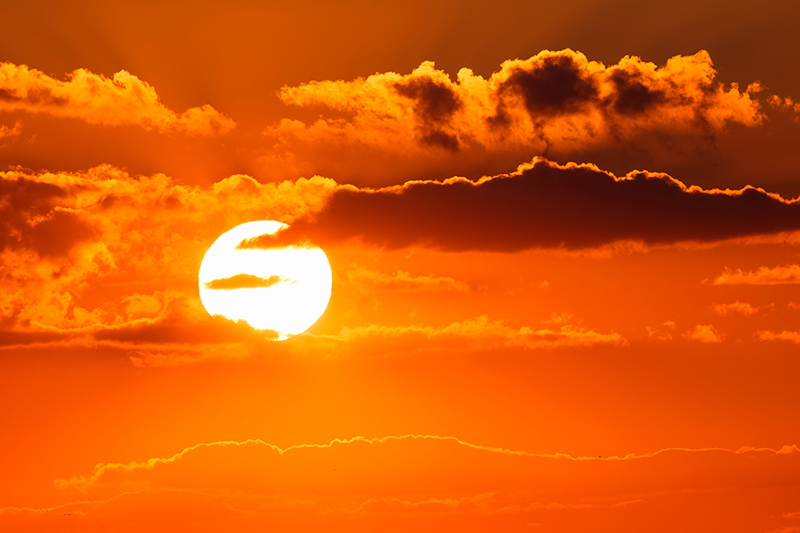This photograph captures a stunning sunset over the water, showcasing a breathtakingly vibrant and almost monochromatic orange sky. The top of the sky transitions from a burnt brownish-orange to a brighter, richer orange with brown undertones as it moves closer to the horizon. A perfectly round, bright white Sun with hints of yellow sits near the horizon, unobstructed except for a few clouds. These clouds range in color from the same deep orange and yellow hues of the sky to darker, more ominous gray and brownish tones. The image appears to be professionally taken, with impeccable quality that makes it frame-worthy. At the bottom of the photograph, gentle waves are visible, indicating the presence of water in the foreground, enhancing the coastal ambiance of the scene. This rich, warm palette and the high-quality capture combine to make a visually striking and beautiful image that epitomizes a serene, picturesque sunset.